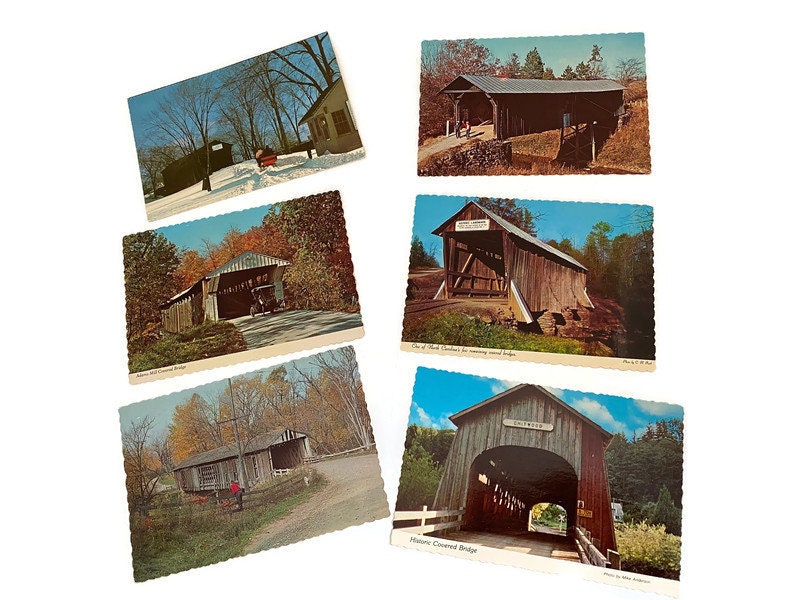The image is a detailed collage of vintage postcards featuring wooden covered bridges in various settings. Each of the six postcards captures a unique bridge scene, portraying the charm and history of these structures. Starting with the top left, there is a wintery bridge scene with a horse and buggy approaching through the snow. Adjacent to it is a long, weathered bridge surrounded by forest and shrubbery. The top middle postcard showcases an antique car driving through another covered bridge, highlighting its historical significance.

In the center, there is a rustic bridge with a person nearby, accompanied by wooden fencing that accentuates its old-world charm. Below it, a bridge spans over water where people are standing, suggesting it might be a pedestrian-friendly structure unable to support vehicles. The bottom left features a weary-looking bridge with a dirt road leading into it, resembling a barn in its architecture. Lastly, the sturdiest bridge is located at the bottom right, appearing more recently built with smoother wood construction, and a vintage car traveling through it.

Each postcard is meticulously detailed, with some displaying the name of the bridge on a white band along the bottom edge. The bridges are set against natural backdrops, often surrounded by trees, enhancing the timeless beauty of these wooden structures.